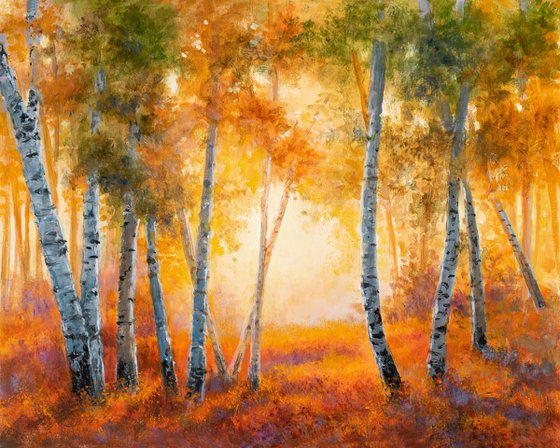This detailed artist's impression, which appears to be a hand-painted representation of a forest, unveils the serene beauty of nature in fall. The painting showcases thin tree trunks, resembling birch trees, with their characteristic narrow, off-white, and gray bark adorned with intermittent black splotches. These trees stretch upward, with the left side densely populated, displaying eight trees, some crisscrossing, while the right side features fewer trees that gradually enlarge towards the center. The foliage, concentrated in the upper halves of the trees, is a vibrant mix of greens, yellows, oranges, and browns, indicating the autumn season.

The forest floor is covered in thick grass, tinted with an orange-yellow hue and highlighted by a subtle purple undertone, further emphasizing the fall ambiance. The background glows with a bright yellow light that dulls into mid-to-light orange tones towards the front, giving the sense of a sunlit clearing at the painting's center. This bright central area creates a pathway-like space, suggesting a hidden destination enveloped in radiant light, adding depth and intrigue to the natural scene.